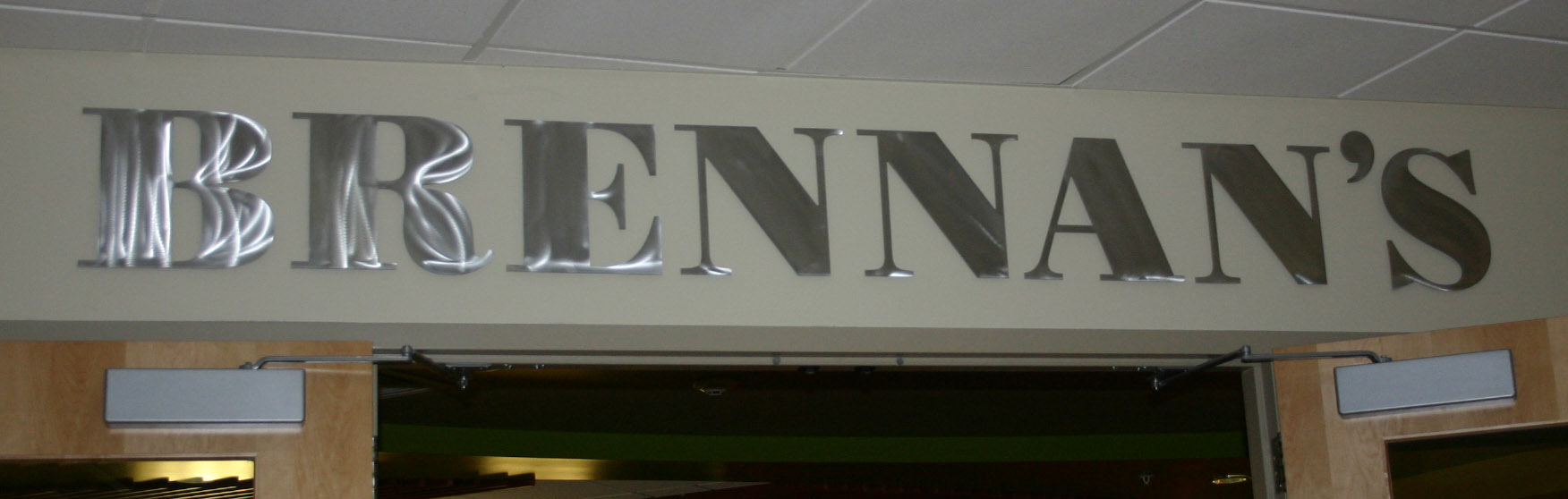This rectangular photograph captures the entrance of a store named Brennan's, displayed in large silver letters on a wall positioned above a double-door entryway. The wall itself is a cream-greenish color. Only the upper section of the doors and entrance area is visible, as the photo is cropped below the Brennan's sign. The double doors are brown with windows and equipped with metal mechanisms to help them close slowly. One door is open, revealing a dark interior space with no visible lighting. The ceiling above consists of white ceiling tiles, and the partial view into the room through the doorway suggests a sizable gap, but details are obscured due to the darkness inside.